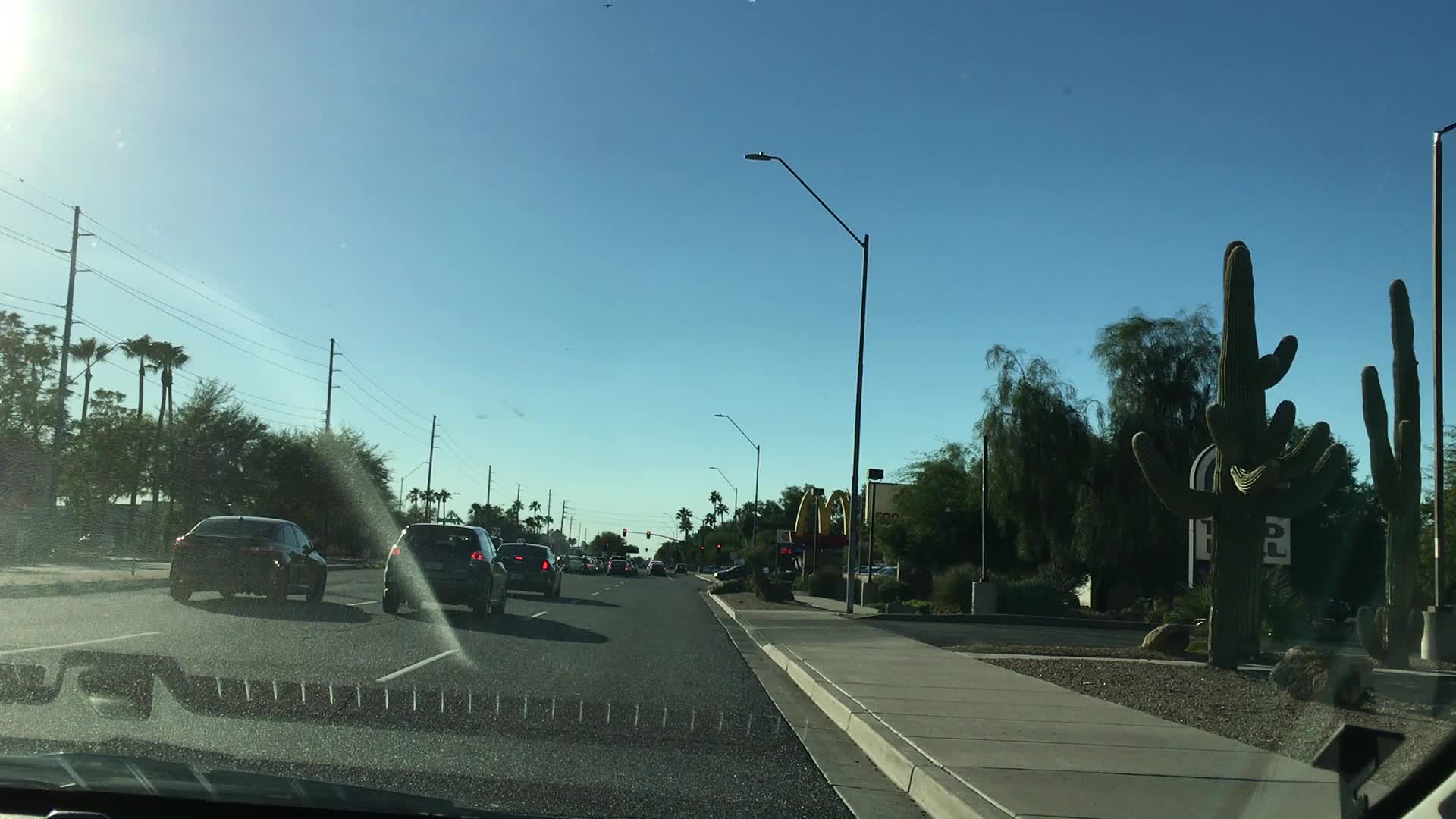This image, captured from a dash cam, presents a clear blue sky with only a single cloud in the top left corner and a bit of the sun peeking in. The bottom half of the image shows a dark black three-lane asphalt road with white lane markings. To the left of the road are power lines and some trees. On the right side of the road, a light gray sidewalk runs adjacent, beyond which is a gravel area with large, tall cacti. Notably, there is a Taco Bell sign behind one of the cacti and a McDonald's sign in the distance with the iconic golden arches. Thin, black-framed street lights line both sides of the road. Several vehicles are visible in the left lanes, driving away from the camera.